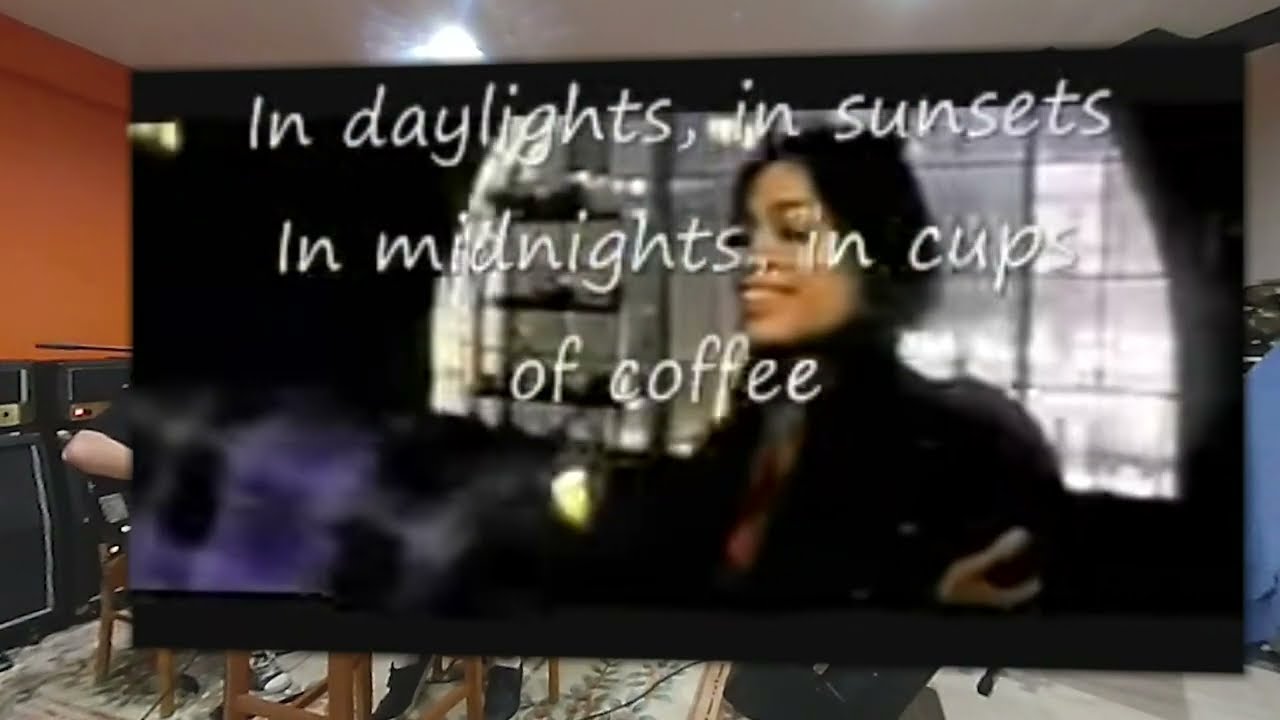The image shows a TV screen displaying a close-up of a smiling Black woman with black hair, wearing a black top or garment with a hood. Superimposed on the screen in white italic script are the words: "In daylights, in sunsets, in midnights, in cups of coffee." The TV appears to be set in an indoor environment that resembles a kitchen or a lounge area. In the background, visible behind and beneath the screen, you can see a table and chairs on a white carpet patterned with green, leaf-like designs. There is a person seated at the table, identified only by their right arm in a black shirt. On the left side of the room, there might be washing machines, suggesting the setting could be a laundromat. The room features an orange wall, shelves, windows, a white ceiling with a lighting fixture, and a mix of furniture and objects that include hints of blue and beige colors.